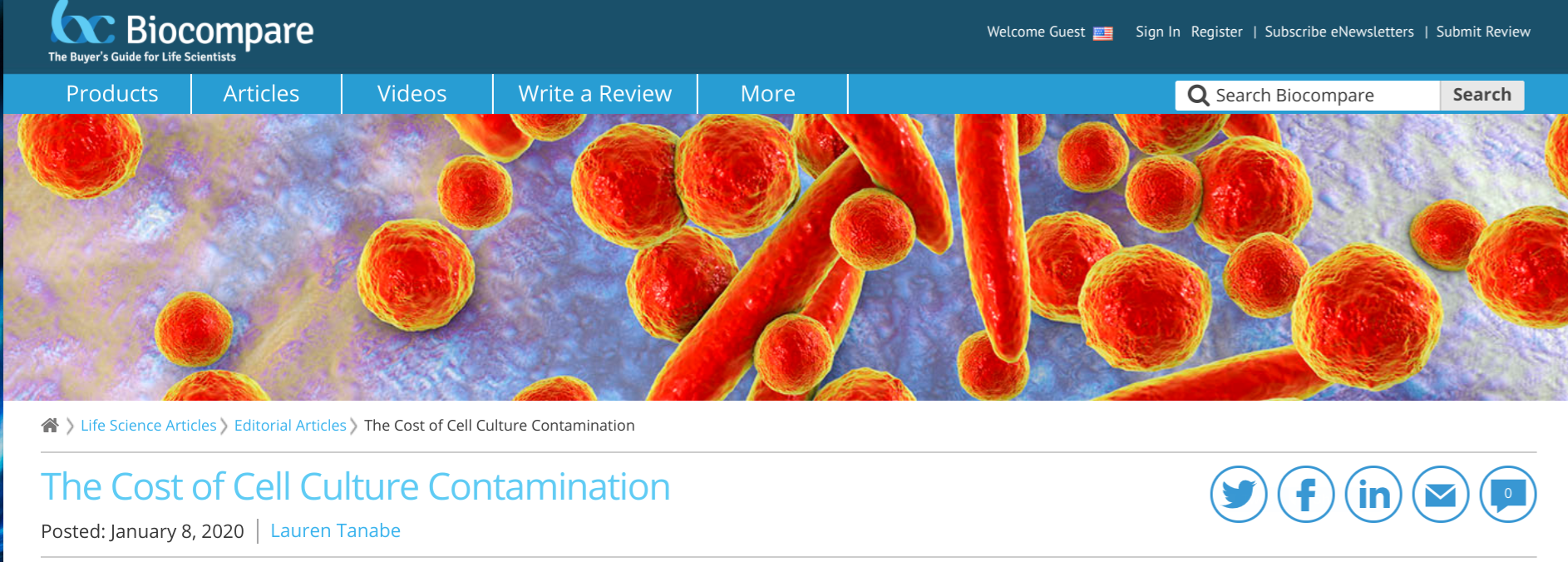This image showcases the homepage of the Biocompare website. At the top left corner, the Biocompare logo is prominently displayed, featuring a blue infinity symbol beside the word "Biocompare." Moving towards the right, the header includes a "Welcome Guests" message accompanied by an American flag. Adjacent to this are links for "Sign In," "Register," a vertical separator, followed by "Subscribe" to the e-newsletter, and finally, "Submit Review."

Beneath this header, there is a navigation bar in a sky blue banner, displaying tabs for "Products," "Articles," "Videos," "Write a Review," and "More." Centrally on this bar, there's a search box labeled "Search Biocompare," with a search button immediately to its right.

Below the navigation bar, the main section of the page features an image that likely represents bacterial or cell cultures, depicted as orange circular and elongated structures. Accompanying this image is a headline reading, "The Cost of Cell Culture Contamination," with an article date posted in January 2020. On the far right side of this section, there are icons for various social media platforms.